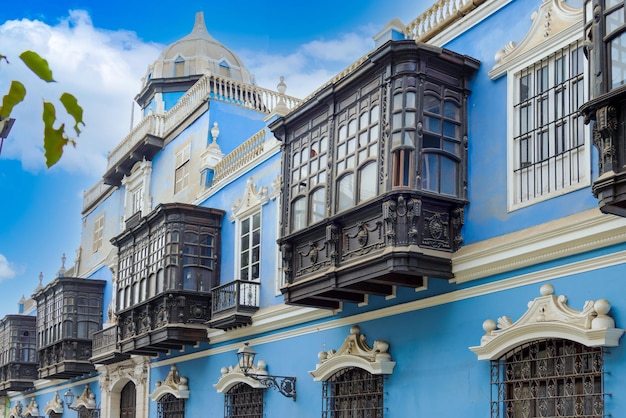The photograph captures a vivid outdoor scene in an urban setting, featuring a prominent building that spans from the left to the right of the image. The building, which appears to be a large structure and might even resemble a castle, displays a striking turquoise blue color with white trim, while parts of its facade exhibit a dark charcoal gray, metallic exterior. Several balconies are visible on the second story, adding architectural interest. The background is dominated by a bright blue sky and scattered white clouds, enhancing the daytime ambiance. In the top left corner, green leaves are caught in the wind, adding a dynamic element to the composition. The color palette includes light blue, black, yellow, beige, white, green, dark gray, brown, and red, contributing to the detailed and rich visual appeal of the urban landscape.